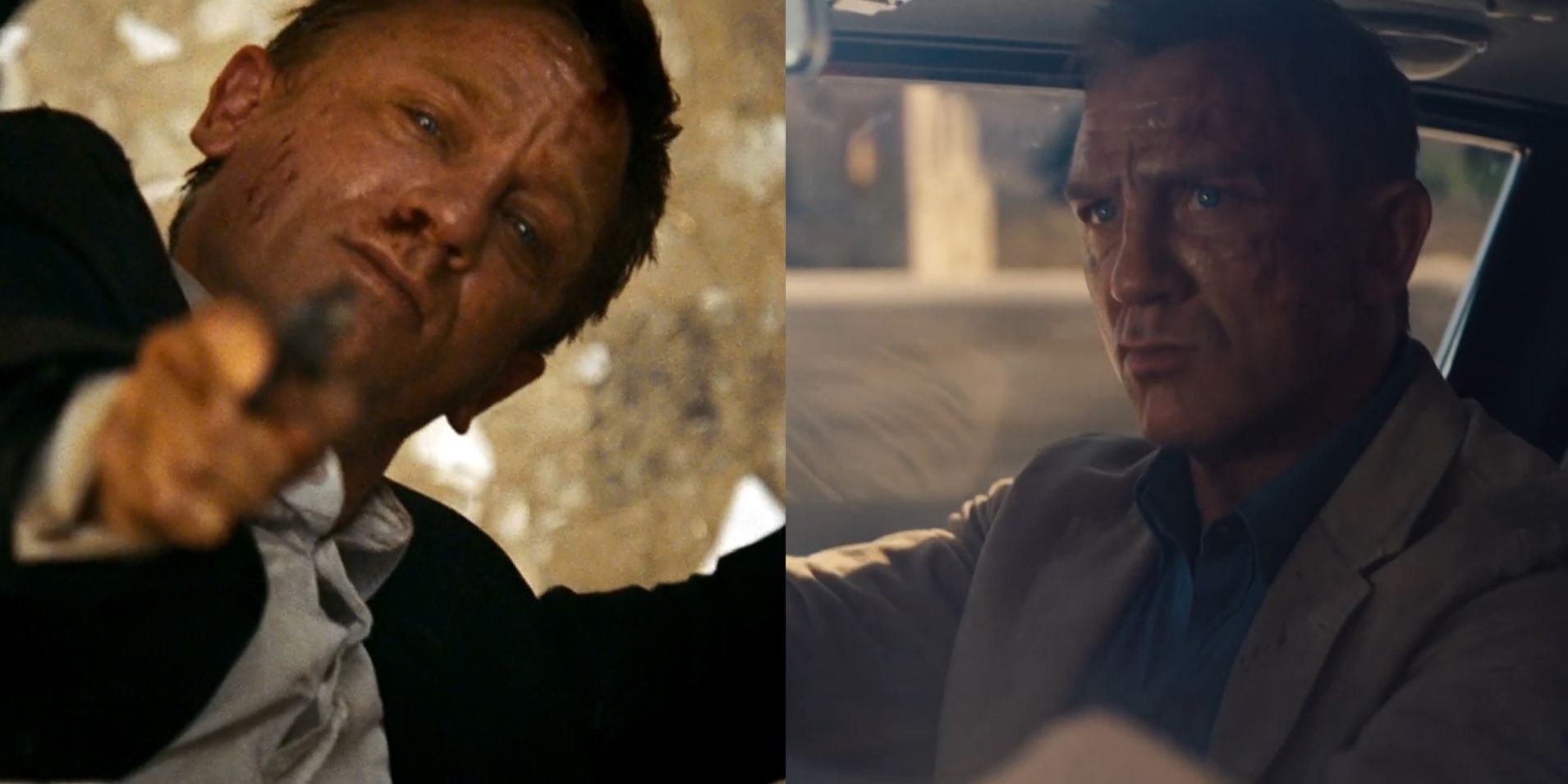The image is a side-by-side composition of two intense and dramatic movie scenes. On the left, a close-up shot captures a man with short dark hair, dressed in a dark suit jacket and a white button-down shirt. His face is dirty and shows signs of struggle, including a bloody nose, suggesting he might have been attacked. He's pointing a gun directly at the camera with a determined, stern look on his face, with a slightly blurred hand and what appears to be a natural, possibly wooded, backdrop.

The right side of the image features another man who bears a striking resemblance to the first but is likely a different individual due to their different hairstyles. This man is seated inside a car, staring intently to his left, possibly at an off-frame subject. He wears a sport coat that could be gray or tan paired with an open-necked dark blue shirt. His face appears sweaty and dirty, contributing to the gritty, high-stakes atmosphere. Both photos are visually dark and convey a sense of urgency and tension, typical of a spy or action film.